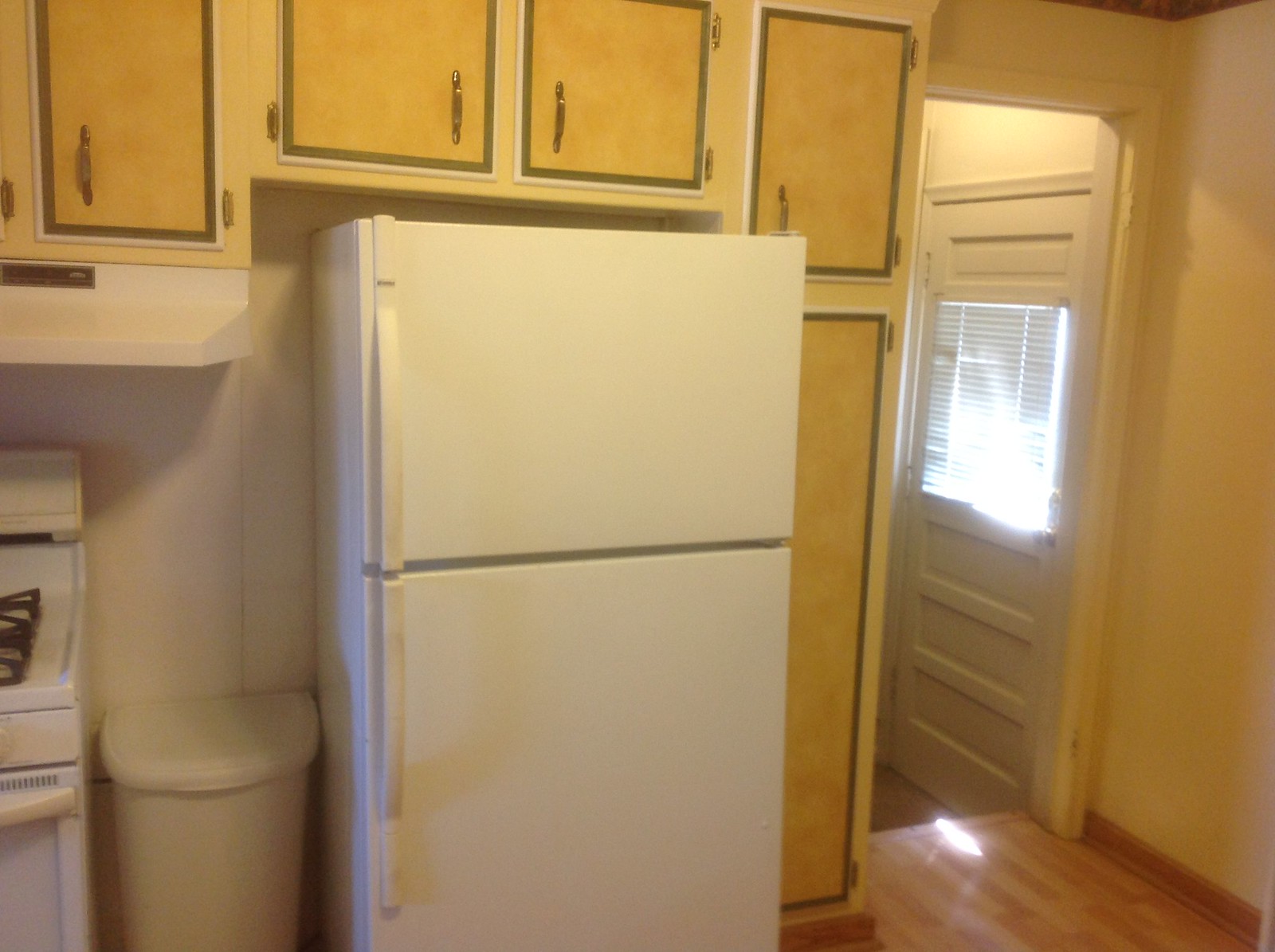The image depicts an older-style kitchen, possibly from the 1970s, characterized by its distinct and somewhat dated elements. Central to the scene is a typical white refrigerator with a freezer compartment on top and a slightly yellowed door, indicating its age. To the left of the refrigerator stands a white trash can, with a gas stove and oven further to the left, showcasing visible burners on the stovetop. Overhead, an exhaust fan is integrated beneath a series of light brown or tan cabinets that frame the refrigerator. These cabinets have metal handles and are embellished with segmented panels, enhancing their vintage appearance. The kitchen floor comprises a light wood laminate, contributing to the overall warm tone of the space. To the right of the cabinets, there is an open doorway leading to a hallway, where another white door with a small window covered by blinds suggests an exit to the outside. The walls of the kitchen are painted white, complementing the light and neutral color scheme of the room.